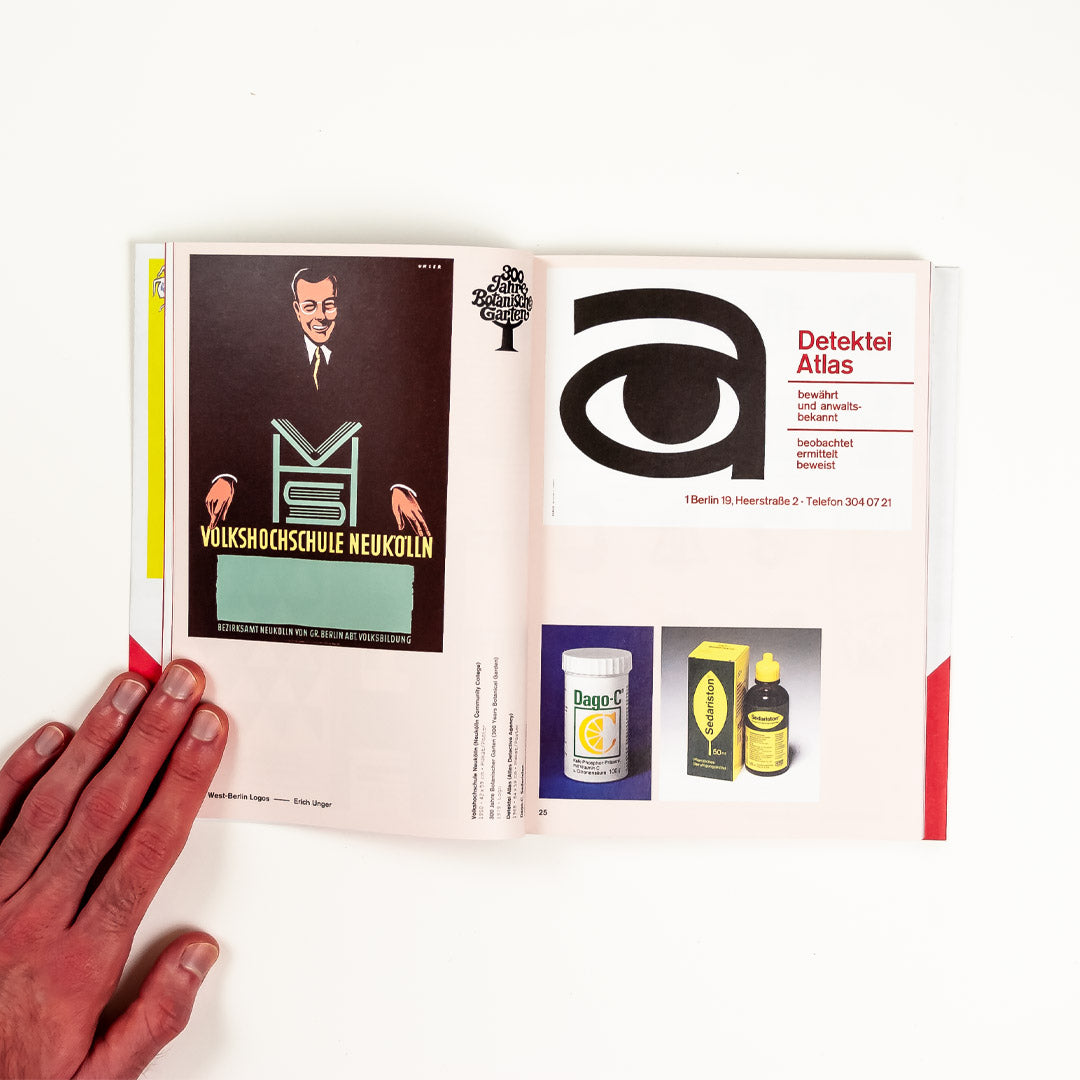In the image, we see an open magazine or book showcasing both the left and right pages. A hand with long fingers, noticeable knuckle hairs, and a reddish complexion holds down the pages from the bottom left. The hand's fingernails appear bluish-silver. The pages of the book are light pink in color.

On the left page, there is a large black rectangle featuring the image of a man who is smiling. His face and both hands are visible, and between him, there is a logo with some letters. The man appears to be standing behind a podium reading from a book, and to his right, there is a sketched image of a tree. The collective text on this page might be written in German.

The right page prominently says "Dekitae Atlas," with an 'I' inside the round part of a lowercase 'a' in "Dekitae". Below this title, there is further information about the atlas. Towards the bottom of this page, there is a collection of items including a white pill bottle, a yellow and gray box, and another yellow and black bottle.

The detailed scene captures the unique textual elements along with the distinct visual details of the hand and the illustrated content on both pages.